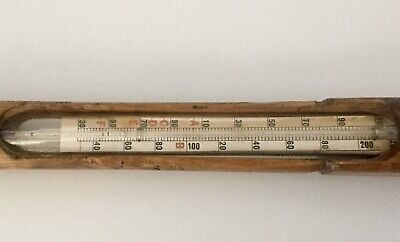This image features an antique mercury thermometer encased in a light wooden shell, exuding an old-fashioned charm. The thermometer is positioned horizontally against a light lavender background, with the bulb end on the left and the top on the right, although it is meant to be hung vertically on a wall, likely outdoors. The thermometer displays measurements in both Celsius and Fahrenheit, ranging from 30 to 200 degrees, with markings on both sides of the glass tube. Notably, the thermometer includes red capital letters from A to F, whose purpose remains unclear but adds to its vintage aesthetic. The wooden casing, slightly aged and imperfectly cut, provides a snug and protective housing for the white thermometer.